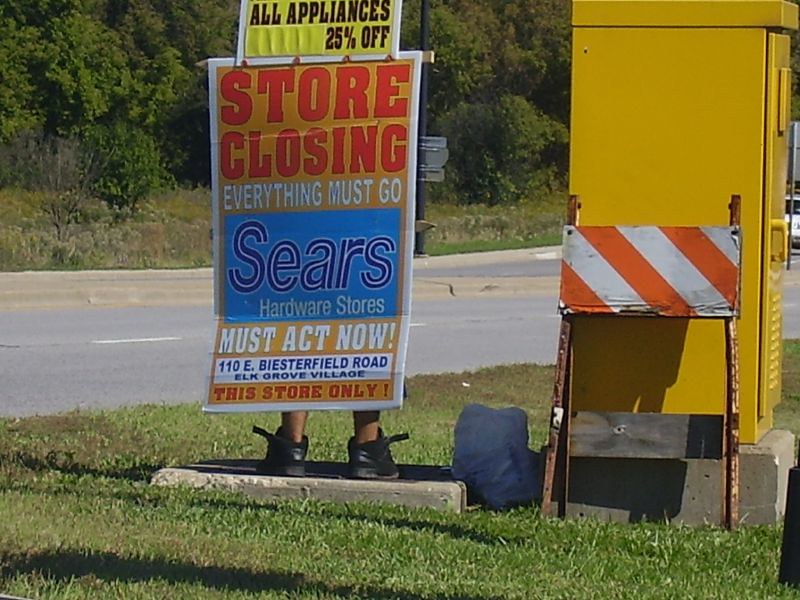In this outdoor photograph, a small highway with a concrete divider runs through the middle, marked by a prominent white line. In the distance, overgrown grass and towering trees frame the road, while closer to the camera, the grass appears more manicured but showing patches of brown. Front and center is a conspicuous store closing sign with bold red letters on an orange background, urgently proclaiming, "EVERYTHING MUST GO" in white. The sign announces the closure of Sears Hardware Stores and instructs customers to "ACT NOW," specifying that this sale pertains to the store located at Elk Grove Village.

Beneath the sign, only the feet of an individual are visible, clad in black shoes, with the person possessing dark skin. Beside them lies a white plastic garbage bag. To the right, on a concrete slab, stands a yellow electrical maintenance booth, accented by a construction sign featuring yellow, orange, and white diagonal stripes, propped casually against the wall. The scene starkly juxtaposes the neglect of the distant overgrowth with the pressing call to action presented by the store's final sale.